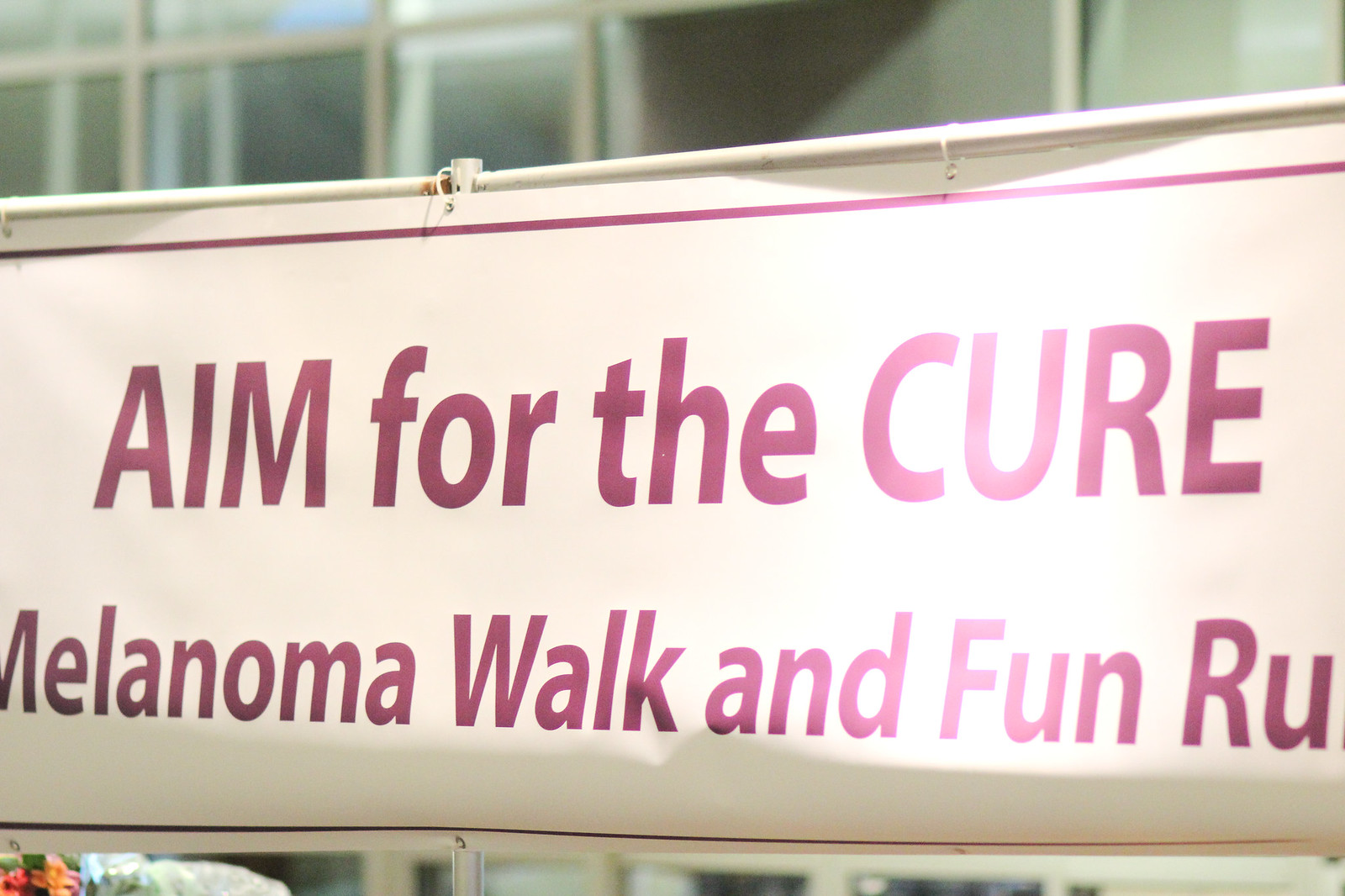The photograph depicts a horizontal, rectangular poster taking up most of the image. The poster is framed at the top and bottom and is affixed with plastic zip ties to what seems to be metallic or plastic bars. The background above shows several glass window panes, suggesting that the poster is likely displayed on a building's wall or doors. The poster features a white background with a bold red border. Within the border, the prominent red text reads, "Aim for the Cure" in very large, uppercase letters. Beneath, in smaller red font, the text states, "Melanoma Walk and Fun Run." Notably, the words "Melanoma," "Walk," and "Fun Run" are capitalized. On the bottom left of the poster, a pink and orange pattern or possibly a flower is visible, although somewhat indistinct. The setting indicates a modern building, likely a mid-20th to early 21st-century structure, given the metal-framed glass panes visible in the upper part of the photograph.